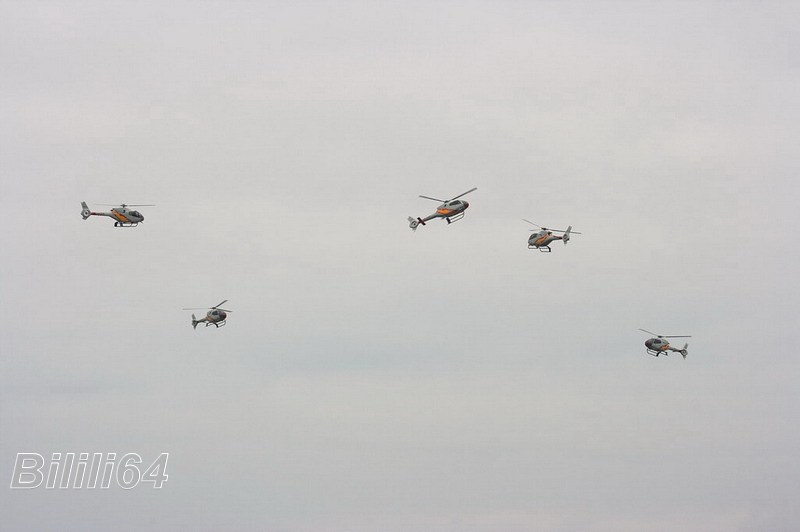The image captures a striking sky setting with a lightly cloudy, grayish-blue backdrop. In the center, five identical small gray helicopters, each adorned with an orange stripe running from top to bottom, are suspended in mid-air. These helicopters are scattered randomly, with their orientations differing; two on the left face inward, one in the middle hovers slightly above facing forward, and the two on the right are directed towards the left. The synchronized elevation of the helicopters accentuates their scattered yet organized appearance. Visible in the bottom left-hand corner, the text "BILILI 64" appears in a clear font, outlined in white, adding an intriguing caption to the composition.